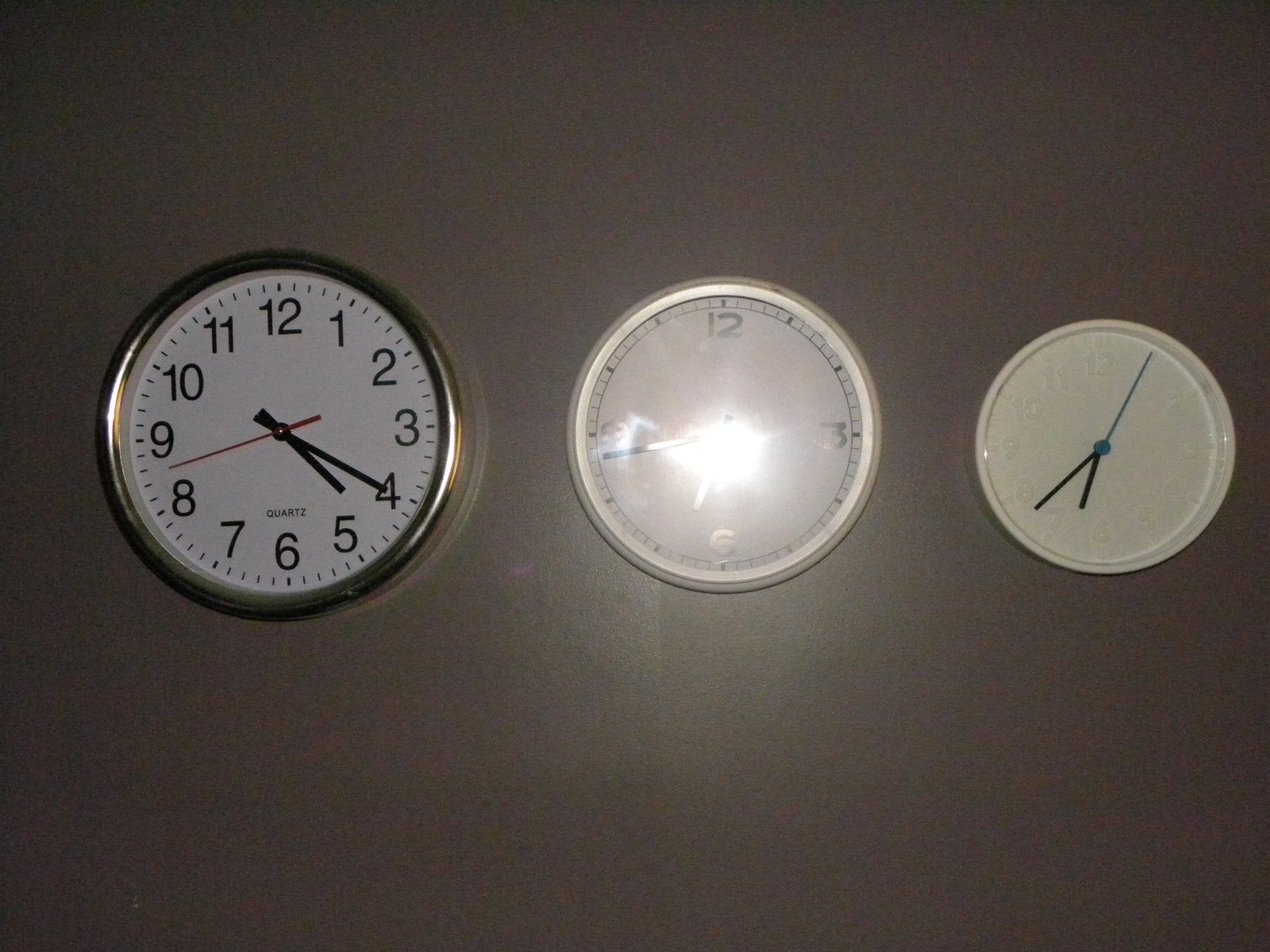A photograph captures a trio of analog clocks mounted on a dark grey wall. The clock on the left, the largest of the three, features a silver frame and is prominently displayed with clear, readable numbers. The medium-sized center clock is partially obscured by a bright glare, likely caused by a camera flash, rendering the 9 almost completely invisible but leaving the 12, 3, and 6 somewhat legible. Finally, the smallest clock on the right boasts a white frame and white numbers, which blend into the background, though the dark blue and black hands remain discernible.